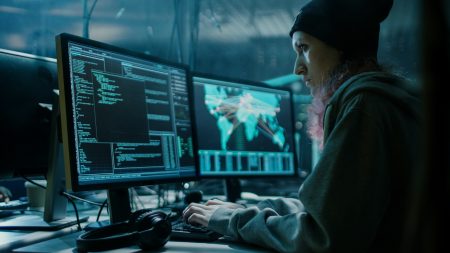In this full-color, horizontally rectangular photograph, seemingly staged indoors under artificial light, the main focus is a woman in her 30s who appears to be a computer programmer or hacker. She dominates the right side of the image, with fairly long, pink hair cascading past her shoulders. She is dressed in a gray hoodie with the hood down, complemented by a black beanie. The setting is a large room with a high, potentially glass-domed ceiling.

The woman is seated at a desk, intently focused on multiple computer screens. She types on a keyboard as she looks at the monitor on her left, displaying a black background filled with green computer code. The right screen showcases a map of North America, South America, and Europe, adorned with red lines and yellow dots, possibly signifying some form of data points or tracking. In front of her on the desk lies a pair of black headphones that she is not wearing. The overall ambiance is framed by gray surroundings, adding to the tech-centric atmosphere of the scene.